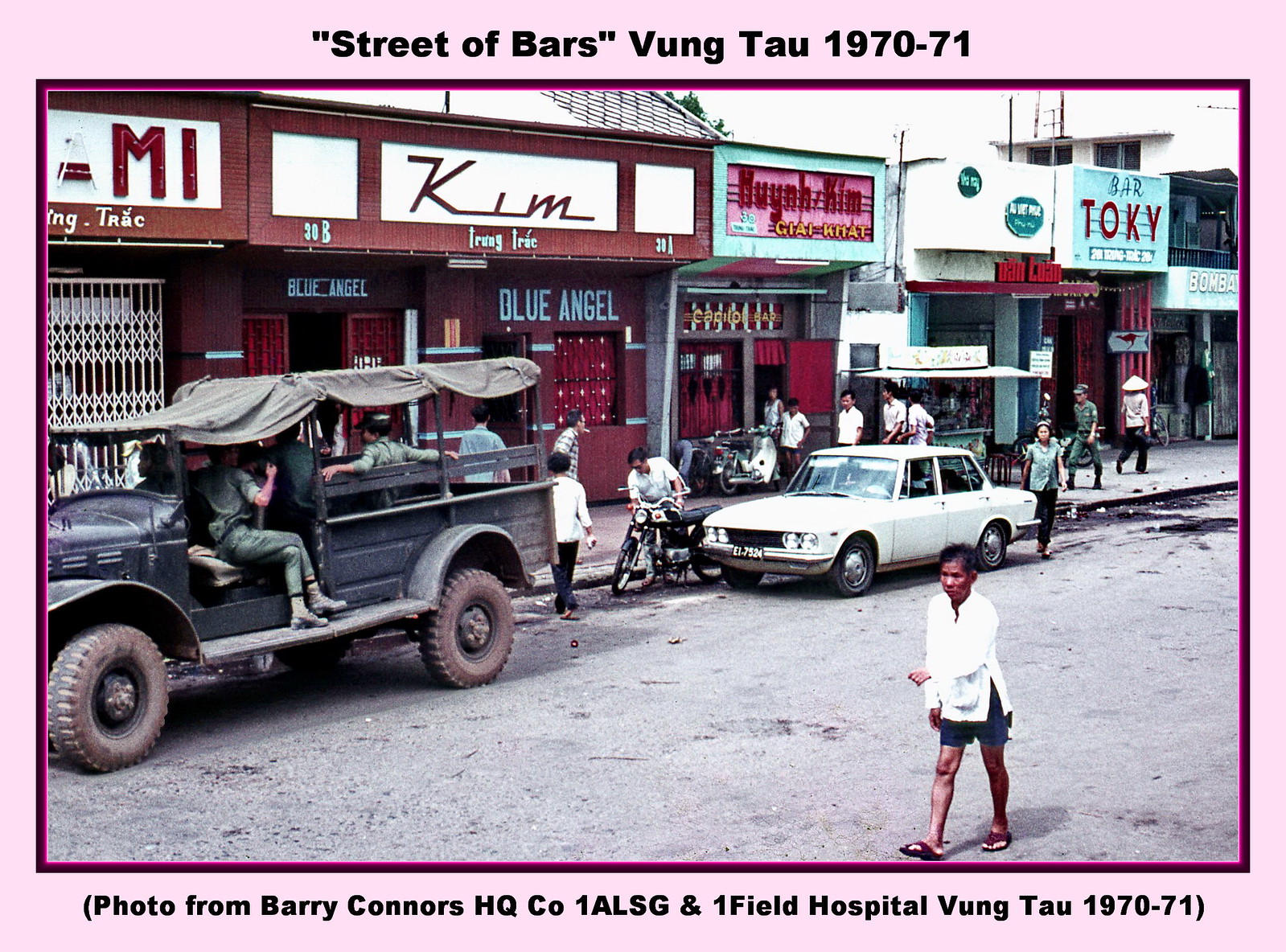The image features a bustling street scene in Vung Tau, Vietnam, during the years 1970-1971. The picture is bordered in pink with black lettering at the top that reads, "Street of Bars, Vung Tau 1970-71." At the bottom, there is a caption: “Photo from Barry Connors HQCO 1ALSG and 1 Field Hospital Vung Tau 1970-71.” The street is lined with various stores, predominantly adorned in red. Notable establishments include a store with "Kim" in red lettering, another labeled "Slash MI," and a third with a green top that reads "Toki" in red letters. Nestled among these is also the "Blue Angel."

The scene is animated with people walking around, contributing to the lively atmosphere. Vehicles populate the street, including a white car resembling an old MG, a motorcycle, and a Jeep occupied by army men dressed in green outfits. There is also a man standing prominently at the front of the picture wearing a white shirt, shorts, and flip-flops. The vivid activity captures a snapshot of life during this historical period in Vung Tau.